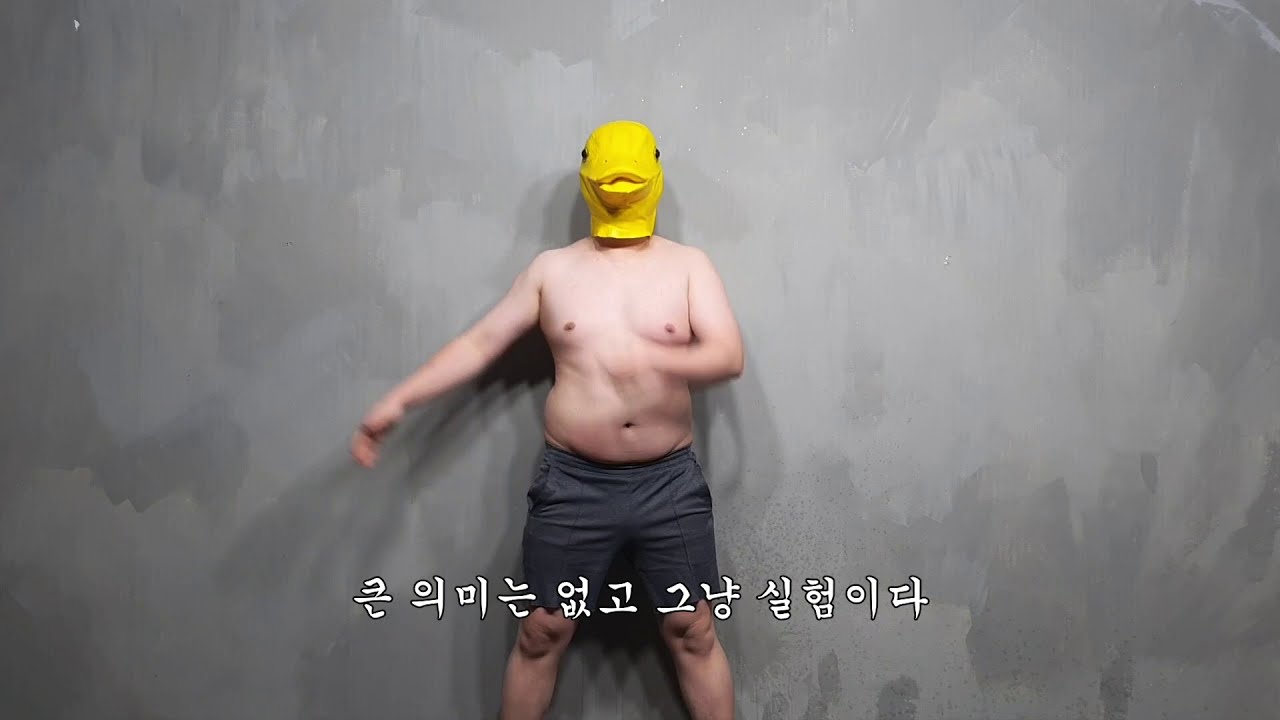In the image, a shirtless, slightly overweight Caucasian man is centered slightly to the left, striking a pose that suggests movement, possibly a dance. He wears tight, dark gray gym shorts and a bright yellow latex duck mask featuring black beady eyes and brownish lips. The backdrop is a blotchy, cement style wall in varying shades of light and dark gray, giving a mosaic effect. His left arm is extended forward, while his right arm, blurred in motion, is bent at a 45-degree angle to the side and downward. Below him, there is some Asian text, possibly Korean or Japanese. The overall scene is humorous and slightly surreal, hinting at a playful or comedic context, such as a photo shoot, TV show, or social media clip.